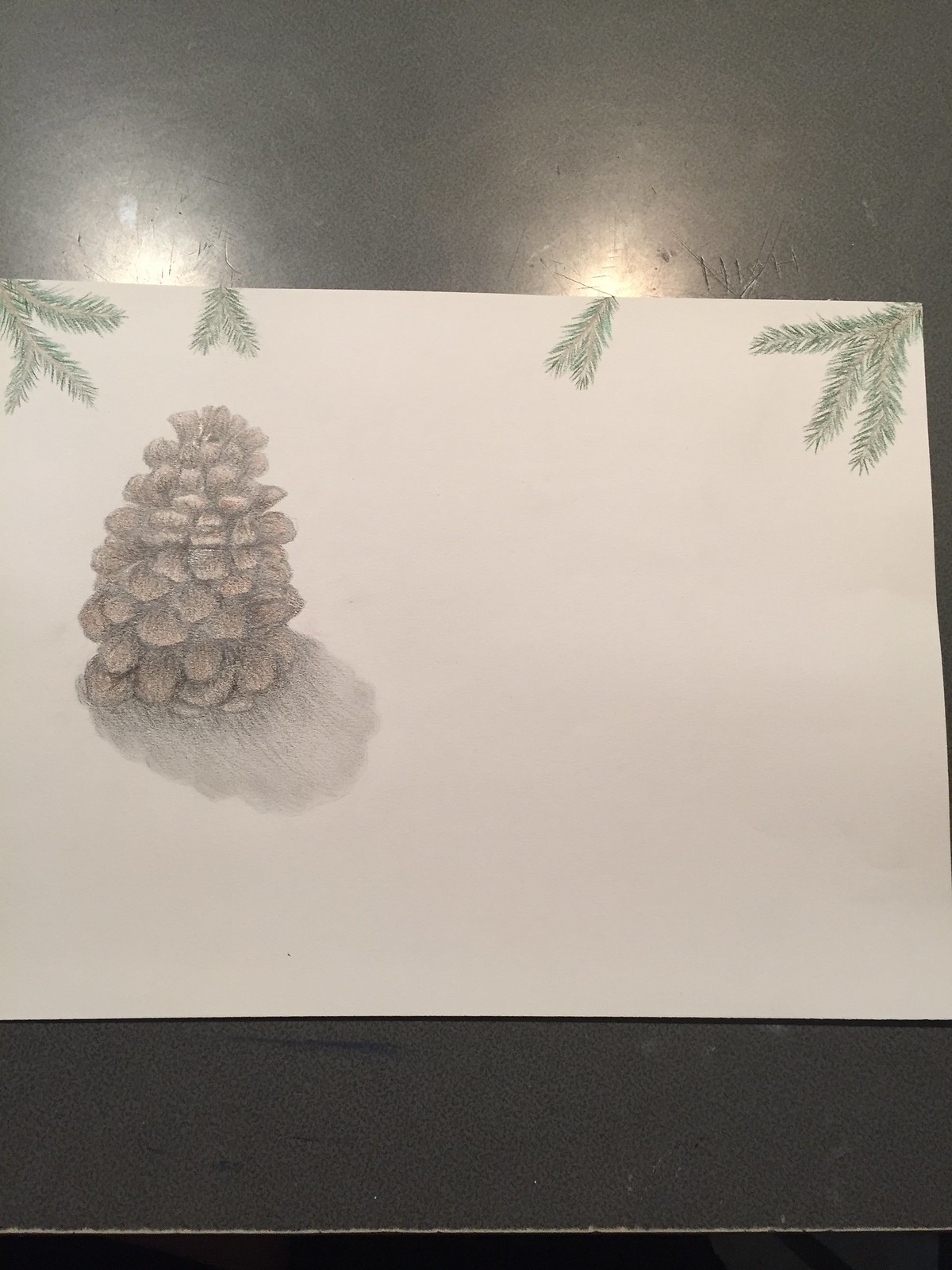The image is a detailed pencil drawing on a blank white sheet of paper. It prominently features a large, vertical pine cone in the middle left, depicted with intricate layers and casting a shadow beneath it. Surrounding the pine cone are sprigs of pine needles and twigs, predominantly located in the top left and right corners. These sprigs are fuller and lush, with multiple clusters of needles and branches adding depth to the composition. The drawing rests on a metallic gray desk that reflects overhead lights, and intriguingly, bears a scratch mark inscribed with the word "NIOH." The overall setup provides a striking contrast between the natural elements of the drawing and the industrial feel of the metallic desk.